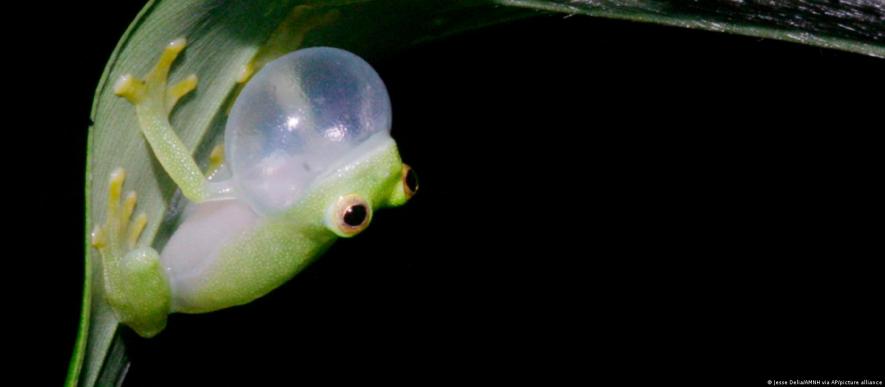In this captivating image, we see a tiny green glass frog clinging to the underside of a curved, green leaf. The frog, almost hanging upside down, is notable for its distinctive appearance; it has a green body with a whitish-gray underbelly. Its throat, expanded into a transparent, bubble-like sac, indicates it is croaking. The frog's large toes, which are a yellowish color, stick firmly to the leaf, demonstrating its sticky grip. The frog's eyes are strikingly large and feature a mix of yellow, black, and reddish hues. The background of the image is dark, adding to the focus on the frog and the leaf. In the upper right corner, a part of a dark green plant is visible, while the overall scene provides no context for the frog’s size. The unique adaptation and features of the frog, such as its glass-like appearance and transparent throat, emphasize its tropical origins and fascinating biology.